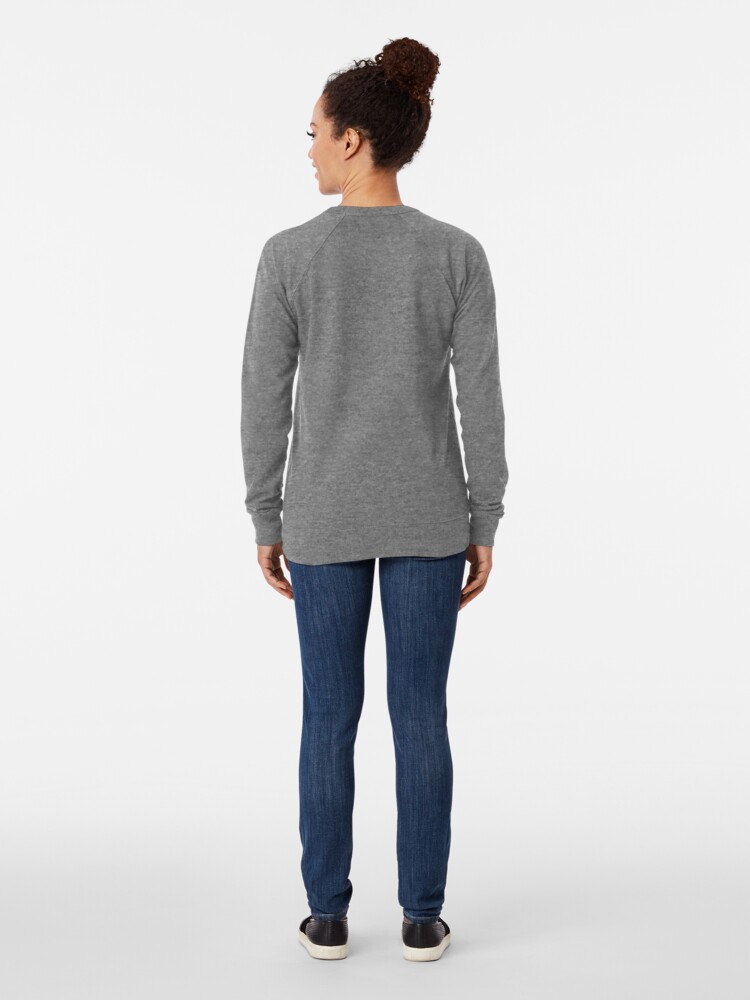In the image, we observe the backside of a human figure standing upright. From the bottom up, we notice that they are wearing black shoes with white outer soles. Above the footwear, blue jeans cover their legs. The individual dons a long-sleeve gray shirt, with both arms resting naturally by their sides. Visible from a side perspective, the hands are relaxed by the hips. The person's neck and head are positioned slightly turned to the left. Their dark brown hair is neatly tied into a bun atop their head. The individual's skin tone is light. The entire scene is set against a plain light gray background, which extends uniformly from top to bottom.